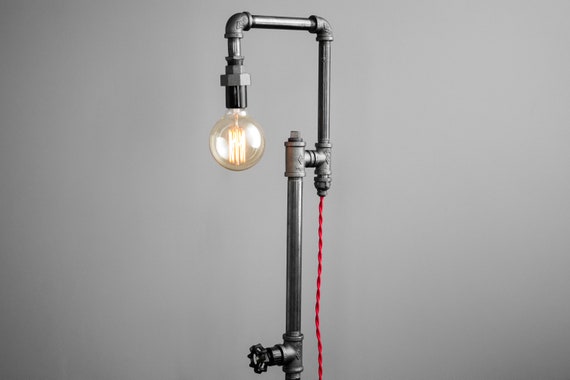This image showcases a unique lamp constructed from metal piping. The focal point of the image is the pipe structure, positioned centrally at the bottom. It includes various segments: a handle at the base, leading into an upward pipe that turns left at an elbow joint and then extends to connect with another pipe. This final segment descends slightly to support a glowing, round lightbulb, highlighting the filament within, which emits a warm yellow-orange glow. The scene is set against a backdrop of empty grayness, accentuating the industrial aesthetic of the pipe-lamp. The colors in the image include shades of yellow, gray, black, and red, with a distinct red line tracing the path of the wiring along the pipe's structure.